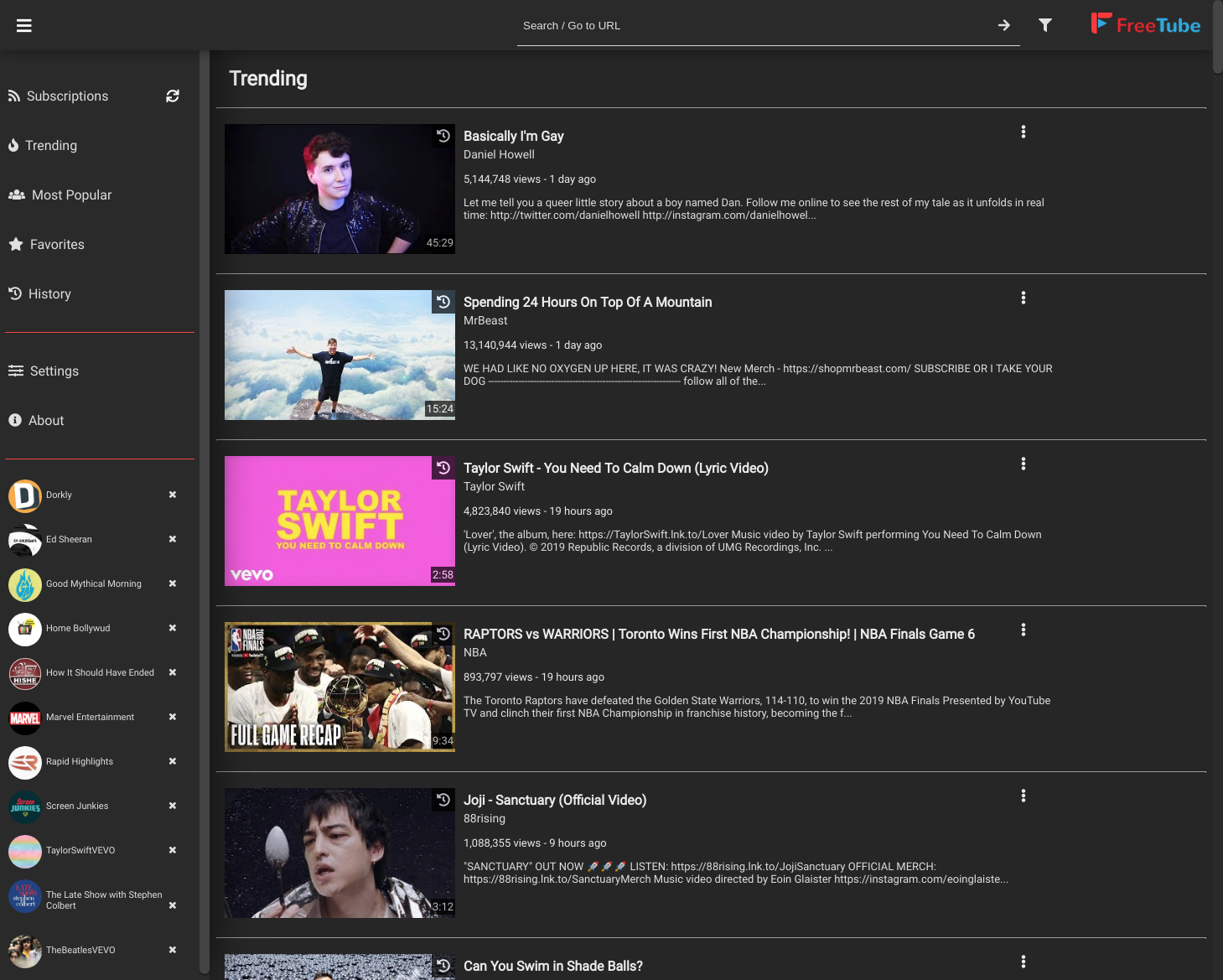Screenshot of the Trending section from FreeTube, a platform resembling YouTube. The company's name, "FreeTube," is prominently displayed in the top right corner. Below to the left is the "Trending" section, showcasing the most popular videos at the moment. The top video titled "I'm Gay" is followed by another titled "Spending 24 Hours on Top of a Mountain." Next, there's a lyric video for Taylor Swift's song "You Need to Calm Down." Additionally, there is a video titled "Raptors vs Warriors: Toronto Wins First NBA Championship, NBA Final Game," capturing the excitement of the historic win. The list concludes with Joji's "Sanctuary (Official Video)," rounding out the diverse range of trending content.